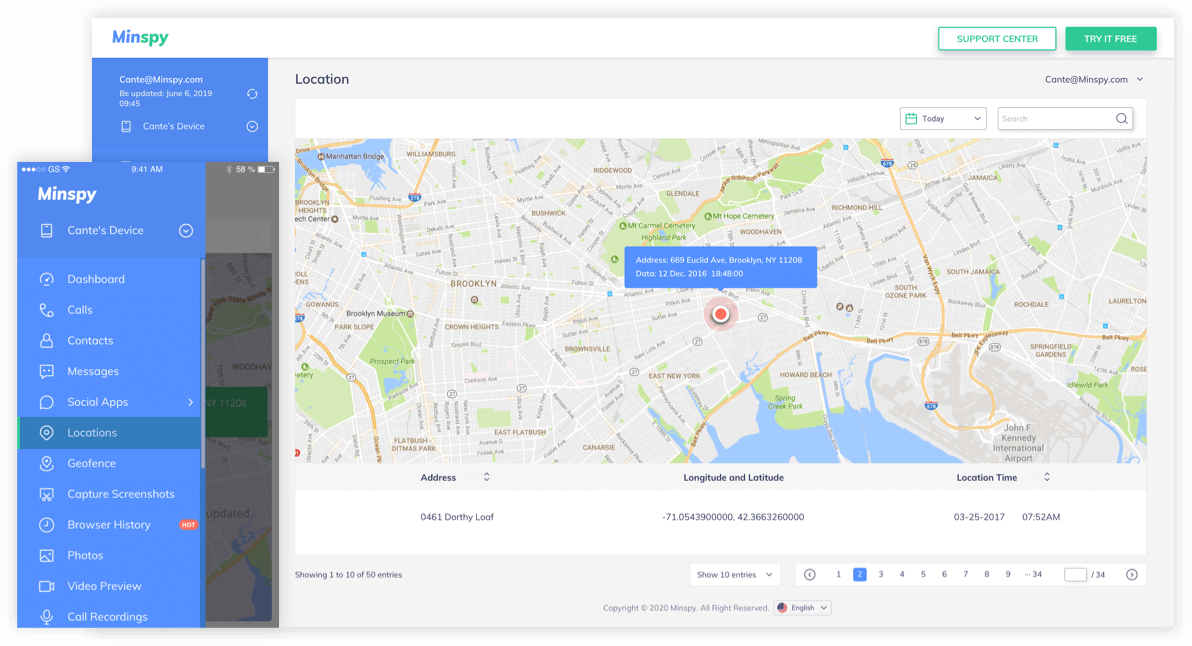The image features a gray background with various elements displayed prominently. In the center, there is a section labeled "Men's Spy" in blue, and "Spies" in green. Below these, there is a green rectangle containing the text "Support Center" also in green. Another green rectangle underneath reads "Triad Free" in white. A map is included, marked with a red circle indicating a specific location. The address and date, "12 December 2016," are provided next to the map. 

In the top-right corner, a green calendar icon displays "Today" alongside a search bar with a magnifying glass icon. At the bottom of the image, the address "010481 Dorothy Loaf" is listed along with corresponding longitude and latitude coordinates, the first of which is negative. Additional details include a time stamp reading "225," the year "2017," and the time "7:52 AM." 

Numbers from one through nine are arranged nearby, with a blue square next to the number two. Following the number nine, a negative value "-34" is shown. To the left, a blue rectangle contains text related to "Men's Speed."